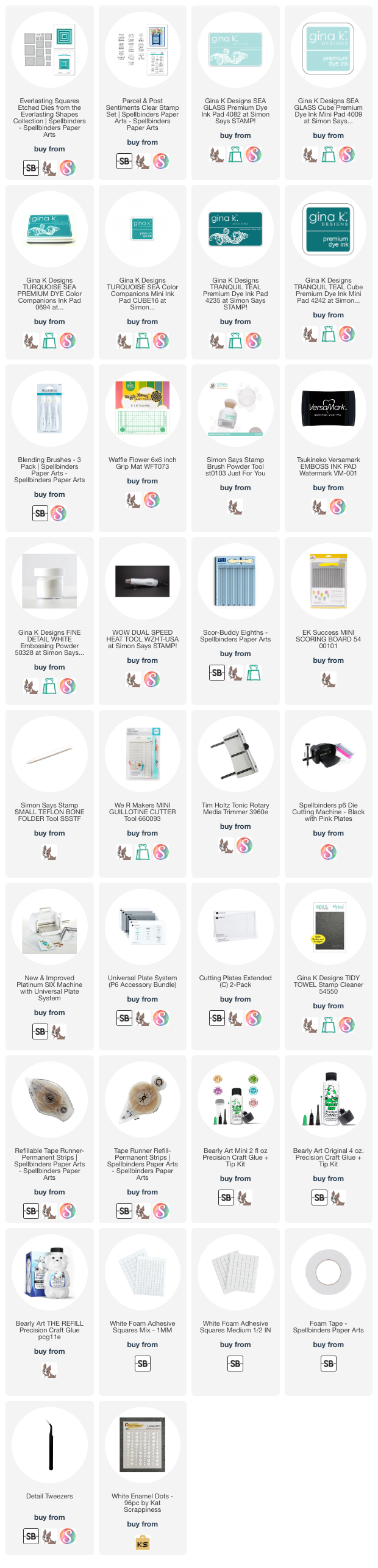A meticulously arranged series of images showcases various purchasable items within a circular layout. Central to the display are the "Everlasting Squares Edge Dies" from the Everlasting Shapes Collection by Spellbinders, prominently encircled. Above this are images of white squares adorned with spirals, available for purchase from SB. One of these squares features a dog's picture inside the letter 'S', consistent across images depicting purchase options.

Adjacent to this setup is the "Parcel and Post" sentiment for clear stamps belonging to the Paper Art Collection. To its right, multiple items from Gina K Designs are displayed, with additional Gina K Designs items spanning across four items per row in a neatly organized grid of nine rows—though notably, the last row contains just two images.

Among the diverse visuals, there's one featuring a pug image, whose purpose remains unclear yet curiously intriguing, alongside another resembling a shopping bag. Each box exhibits a subtle gray hue with a circularly shaped image inside, providing a brief description and purchase instructions.

The arranged display aims to inform viewers about the available products, offering details on where and how to buy them.